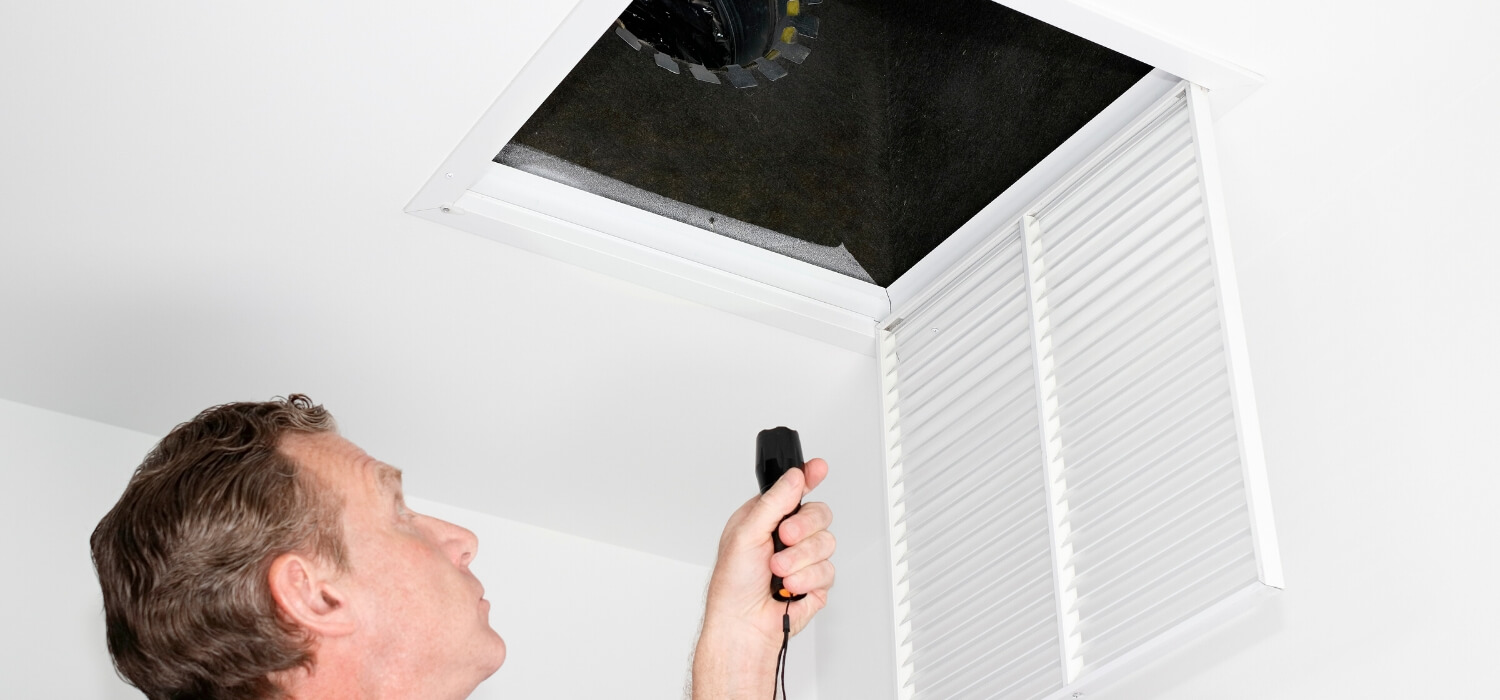In this detailed, full-color indoor photograph, a middle-aged white male with short, wavy brown hair is captured inspecting a ceiling vent. The surroundings are simple, featuring white walls and a white ceiling. The vent's grate has been removed and is hanging down, revealing a dark, black void within the ceiling. The man, visible from the right side and extending up to his neck, is holding a miniature black flashlight in his left hand, which has a cord dangling from it. He appears to be thoroughly examining the black area inside the ceiling, likely inspecting an HVAC unit such as an air conditioning or heating system. The artificial lighting in the room highlights the details of this scene, creating a sharp contrast against the dark space within the ceiling.